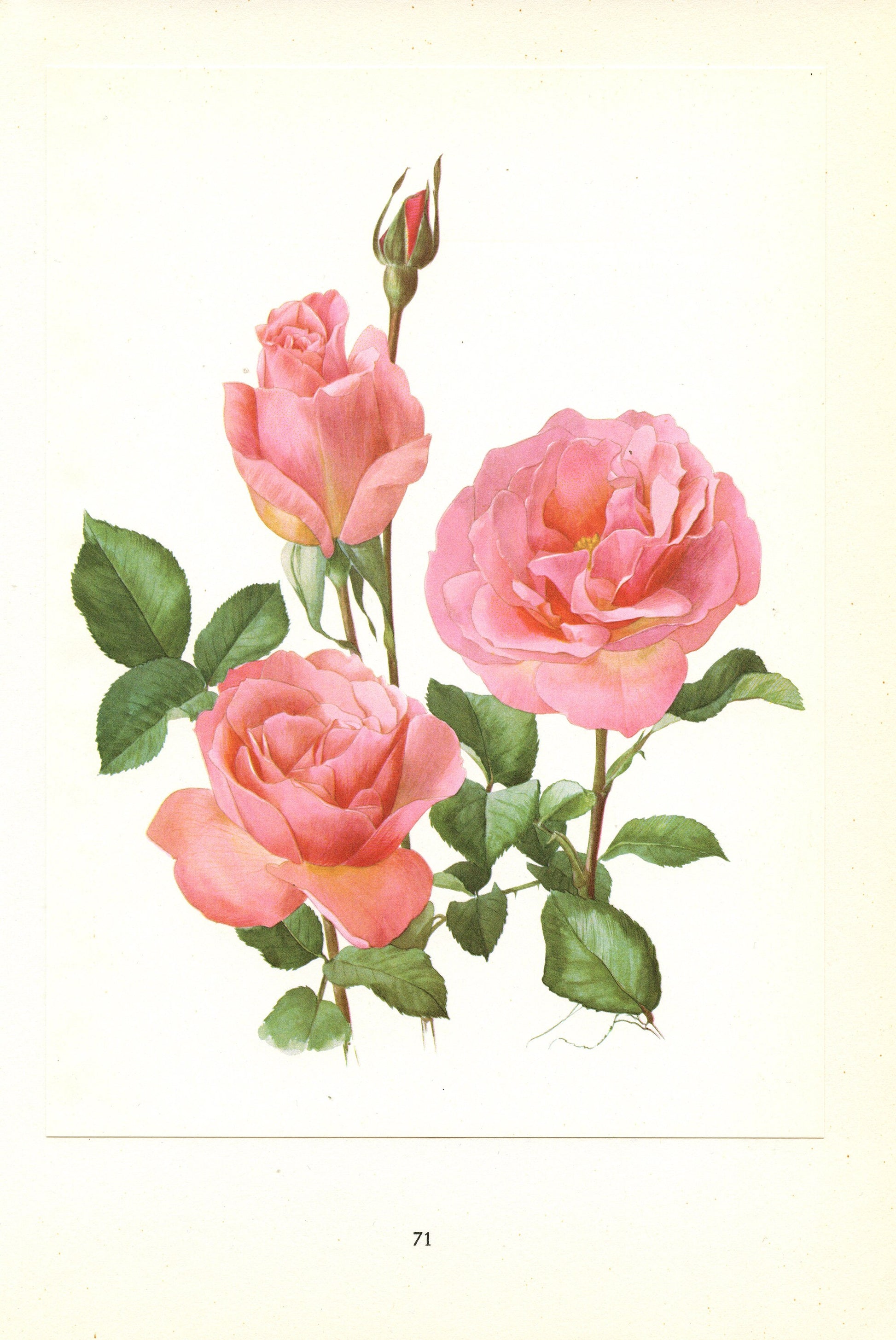The image is a detailed depiction showcasing four pink roses at various stages of blooming, set against a pristine white background. The two fully bloomed roses radiate a vivid pink hue, captivating the viewer's attention. In the upper left, a more youthful rose bud emerges, accompanied by a completely closed bud in the background. The green leaves add a striking contrast, their intricate details and prickly stems enhancing the overall allure. Though described by some as a painting due to its remarkable detail and depth, the image is convincingly realistic, resembling a high-quality photograph. There is no text in the image, but a unique identifier, the number 71, appears near the bottom left, with a light yellow border framing the composition. This beautiful arrangement stands out with its simple yet elegant color palette of pink and green, making it reminiscent of a perfect flower arrangement.